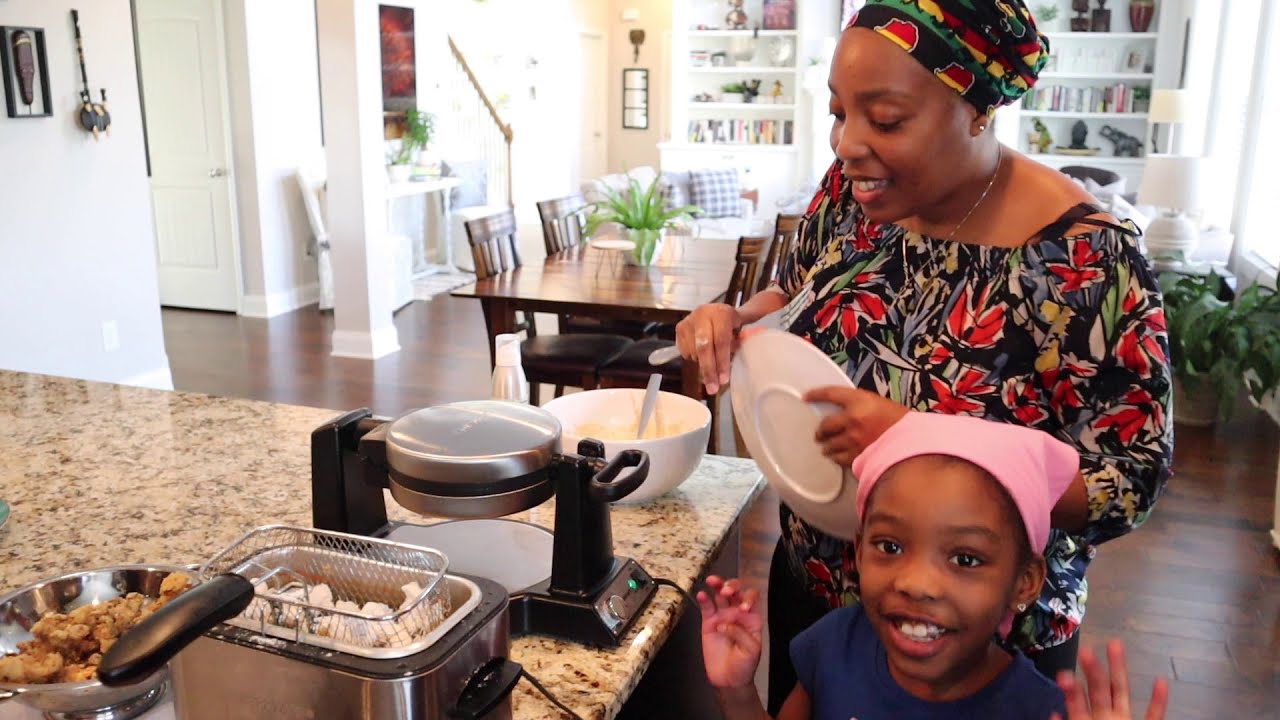In this warm and inviting daytime scene, a mother and her young daughter are seen cooking together in a cozy kitchen, filled with natural sunlight. Positioned to the right side of the wide, rectangular photograph, the mother, a black woman with dark brown skin, is dressed in a vibrant patterned shirt adorned with red, blue, yellow, and green flowers, as well as a matching headdress. She focuses intently on the food in front of her, holding a white plate in one hand. Her daughter, also with dark brown skin and wearing a pink bandana and a blue shirt, stands beside her, hands joyfully raised and smiling directly at the camera.

The kitchen features an island counter laden with bowls of food, while the bottom left corner reveals a glimpse of a marble countertop. In the background, a dining room with a dark brown table set for four is partially visible, along with a living room and a bookshelf area to the top right. Additional homey elements include plants and shelves centrally located behind the mother, further enhancing the sense of a lively, lived-in space. On the left, two hallways and the start of a stairwell with brown railings add depth to the photograph. The entire composition exudes a sense of familial warmth and cherished quality time spent together.